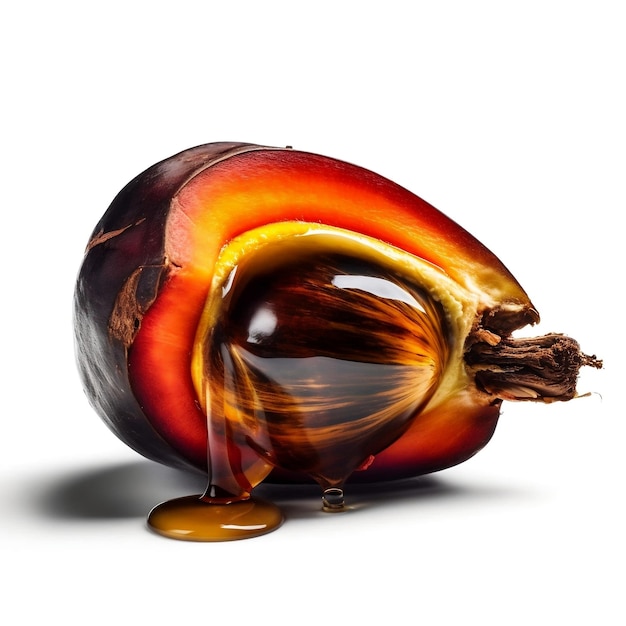This image captures a unique and intriguing fruit that closely resembles the shape of a pear. The skin of the fruit is rough and dark, exhibiting a deep cranberry-maroon hue that suggests aged and decaying, with an old, brittle stem at the top. The fruit has been cut open vertically, revealing a strikingly vibrant interior. The flesh transitions from rich reds and oranges to yellows, resembling the colors of a sunset. Nested at the core is a large, smooth pit or nut about the size of a golf ball, characterized by marbled streaks of deep brown and lighter hazel, akin to a bowling ball. Surrounding the pit is a thick, viscous substance resembling honey or pancake syrup, which is oozing onto the white surface on which the fruit rests, adding a shiny, gleaming texture to the scene. The overall interior texture of the fruit's flesh is somewhat reminiscent of a pomegranate, with intricate layers and a vivid palette.